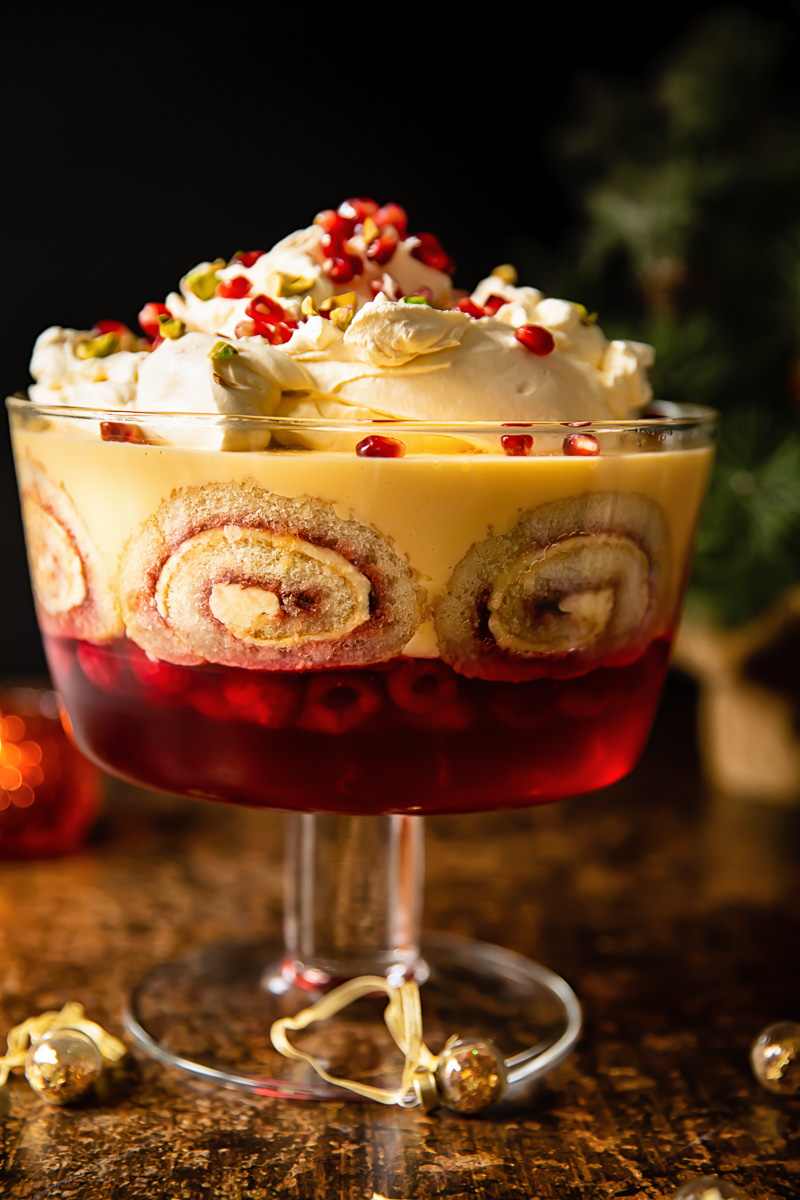The image captures a detailed color photograph of a lavish layered dessert presented in a large, multi-serving trifle dish mounted on a clear glass pedestal. The bottom layer of the dessert features a vibrant red gelatin or raspberry jelly. Above this, there are intricate curlicue slices, perhaps from a rolled cake, embedded in a rich, butterscotch-colored pudding. The top layer is a generous helping of whipped cream, adorned with a sprinkle of pomegranate seeds and chopped pistachios. The dessert is placed on a well-worn, glossy wooden tabletop dotted with festive gold jingle bells on ribbons. In the blurred background, greenish and orangish shapes hint at seasonal decor, while hints of foliage or plants imply an indoor setting.